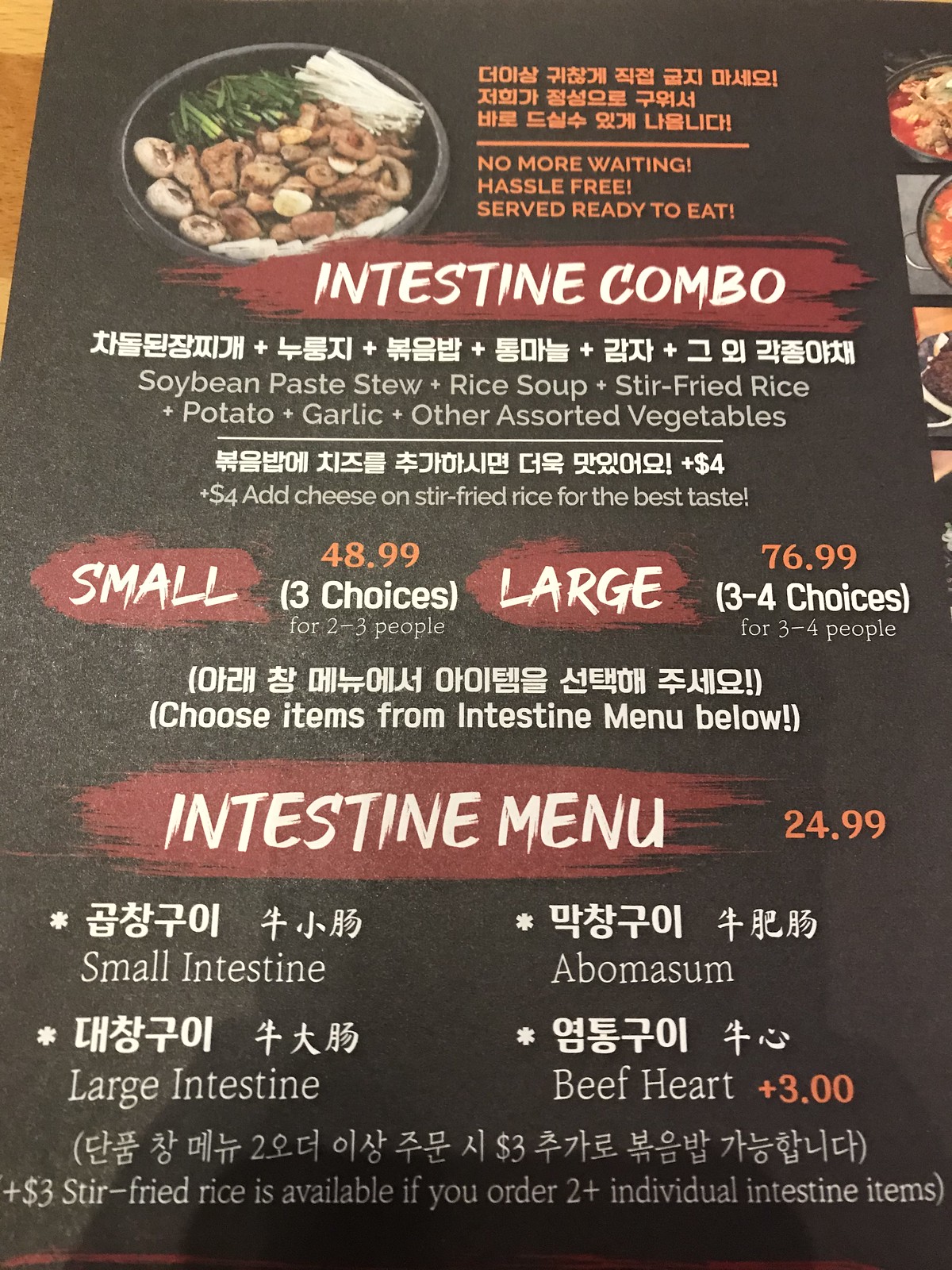The image portrays an intricately designed restaurant menu that presents a blend of English and Korean text. The menu has a sleek black background with vivid details. 

At the top left corner, there is an image of a black dish brimming with an assortment of colorful vegetables including chopped greens, white vegetables, mushrooms, and brown vegetables. Adjacent to the picture, vibrant orange Korean text is displayed alongside an English phrase that reads, "No more waiting, hassle-free, served ready to eat."

Beneath this, within a red paint-stroke border, white text announces, "Intestine Combo." Below this heading, additional Korean writing appears, followed by an English description: "Soybean paste stew, plus rice soup, plus stir-fried rice, plus potato, plus garlic, plus other assorted vegetables." Further down, more Korean text is written in white, stating "+ $4," and then another line informs, "Add cheese on stir-fried rice for best menu."

Continuing down, the menu lists various items, categorizing them between "Small" and "Large" options. The "Small" option is priced at $48.99 and offers three choices, while the "Large" option is priced at $76.99 and provides three to four choices. Below these options, more Korean writing is interspersed with English text instructing, "Choose items from intestines menu below."

This section is bordered by another red paint-like label, which reads, "Intestine Menu." To the right, in bold orange text, the price $24.99 is indicated. The menu then lists several items, first in Korean, and subsequently in English: "Small Intestine," "Abomasum," "Large Intestine," and "Beef Heart." 

At the bottom of the menu, an addendum in parentheses (also in Korean) is paired with an English note stating, "+ $3 stir-fried rice is available if you order two plus individual intestine items."

On the upper right side of the menu, there is a collage of four different, yet slightly cut-off images of menu items, each displayed within small squares.